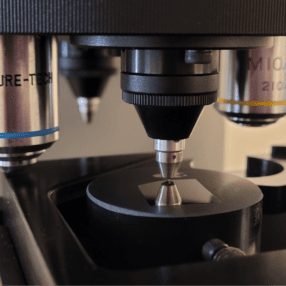This photograph presents a close-up view of the turret lens section of a microscope. The image, which is square and quite small, captures several cylindrical lenses of varying magnifications, suspended from black plastic housing at the top. The lenses, identifiable by their metal tips, almost touch a round glass plate below, which likely holds a specimen. The turret mechanism, enabling lens rotation for different magnifications, is visible, and one lens is marked with the brand name "SureTech," while another has the inscription "MIO 210" with a yellow paint stripe, and yet another shows partial lettering "RETCH" with a blue line.

The photo is taken from an angle that excludes the body and upper lens of the microscope, focusing solely on the interchangeable lenses and their immediate surroundings. The background is a plain white wall with a visible shadow, emphasizing the mechanical details of the microscope against a stark backdrop. The base of the microscope, which is not fully shown, seems to have a small switch or knob in the bottom right-hand corner, adding to the detailed view of the mechanical intricacies.